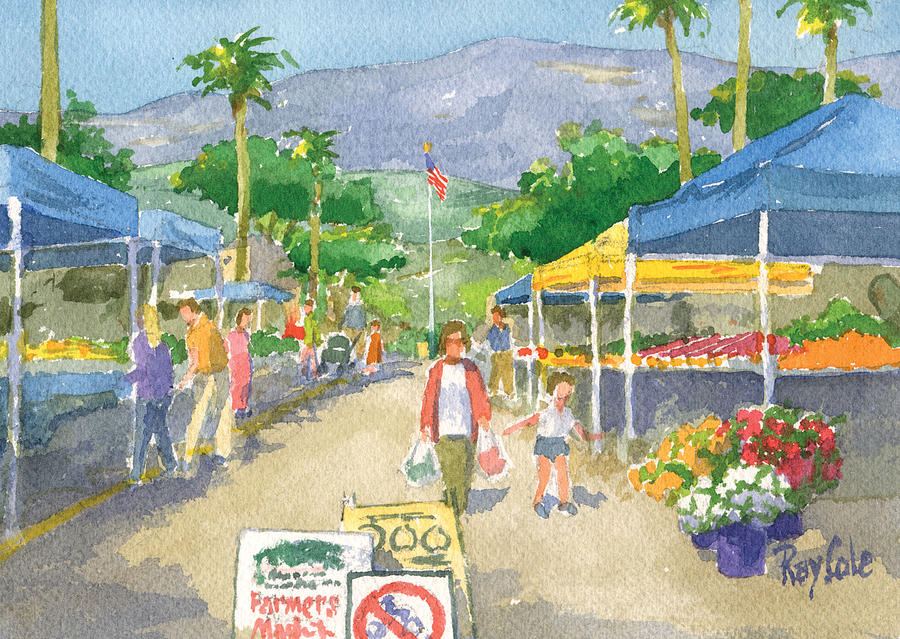The image is a horizontal rectangular watercolor painting depicting a bustling farmer's market, likely set in Los Angeles, given the presence of tall, swaying palm trees. The market's layout includes booths on either side of a central dirt path, each covered by colorful awnings—primarily blue, with a lone yellow awning halfway down the path. In the foreground, a clear sign reading "Farmer's Market" is visible, alongside a caution sign and a no bicycle sign. A mother and daughter are walking towards the viewer; the mother, dressed in a red waist-length jacket over a white blouse and green pants, carries cellophane bags filled with purchases. Her daughter wears a white shirt and blue shorts, skipping by her side.

To the lower right, three pots of flowers bloom with white, red, and orange petals. The booths along the pathway display a vibrant array of produce, including oranges, apples, pumpkins, tomatoes, and possibly peppers. Further down, more shoppers peruse various stands, with the American flag atop a pole drawing attention at the far end of the walkway. The artist’s pastel palette beautifully captures the lively and colorful ambiance of a community gathering spot.